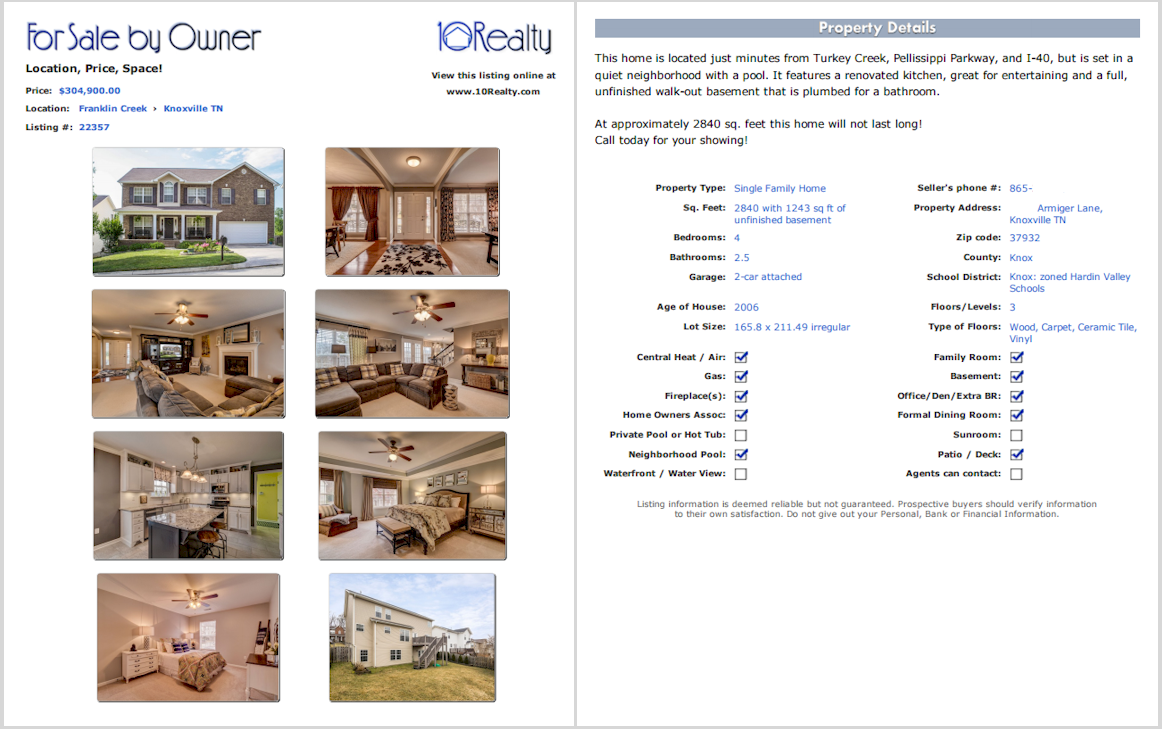For sale by owner: Spacious single-family home in Franklin Creek, Knottsville, Tennessee, listed at $304,900. The listing number is 22357.

On the right side, you can view the detailed property listing at www.1010realty.com presented by 1010 Realty. The property includes four rows of photographs showcasing the home's interior and exterior features. Among these, two photos highlight the exterior, while the remaining images provide an in-depth look at the beautifully designed interior spaces.

Property Details:
- Located just minutes from Turkey Creek, Plessy Parkway, and I-40, set in a peaceful neighborhood with a community pool.
- Features a renovated kitchen perfect for entertaining.
- Includes a full, unfinished walk-out basement that is plumbed for an additional bathroom.
- Total living space of approximately 2,840 square feet.
- The house includes 1,243 square feet of unfinished basement.
- Four bedrooms and 2.5 bathrooms provide ample accommodation.
- Prompt listing: This property is in high demand and won’t last long. Call today to schedule your showing.

Don't miss this opportunity for modern, comfortable living in a prime location.